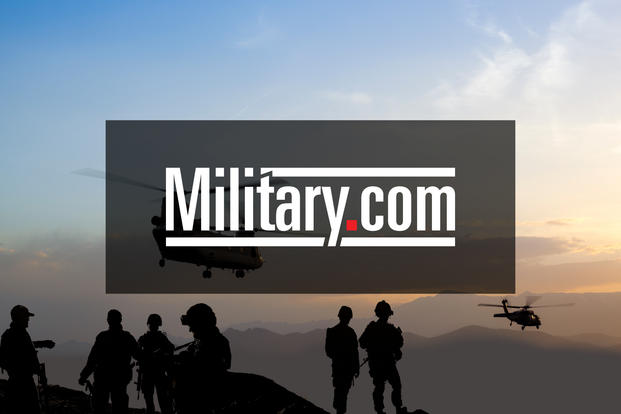This striking image captures a military scene during sunset, prominently featuring a dark gray, transparent rectangle in the center with the white text "military.com" bordered by thin white lines, and a red dot in the website name. The foreground shows six soldiers in black silhouette, most wearing helmets and holding guns, standing atop a mountaintop. To the left, four soldiers cluster together while two stand side by side to the right. The background reveals two dark silhouettes of helicopters—likely Apache helicopters—soaring above the hilly, gray-and-black terrain. The sky transitions from a deep blue at the top to a golden yellow near the horizon, with wispy clouds adding to the dramatic atmosphere. The overall scene suggests a military drill against the stunning backdrop of the mountainous landscape.